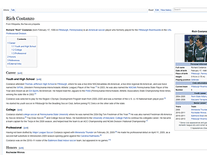The image is a screenshot of a Wikipedia page, likely captured from a PC or laptop. The page features a detailed biography of an individual named Rich, possibly with the surname Colabertre, though the name is somewhat unclear due to blurriness. To the right side of the page, there is a photograph of Rich, along with his date of birth and other personal information, such as likely his place of birth and educational background.

The middle section of the page appears to summarize Rich's career accomplishments, suggesting he may be a sports figure, possibly a basketball player. Although some parts of the text are blurred, sections detailing his major achievements and career highlights are visible, alongside information about his college career and the teams he played for. Despite the brevity of the page, it meticulously outlines key aspects of Rich's professional journey, offering a comprehensive overview of his contributions and milestones in the sport.